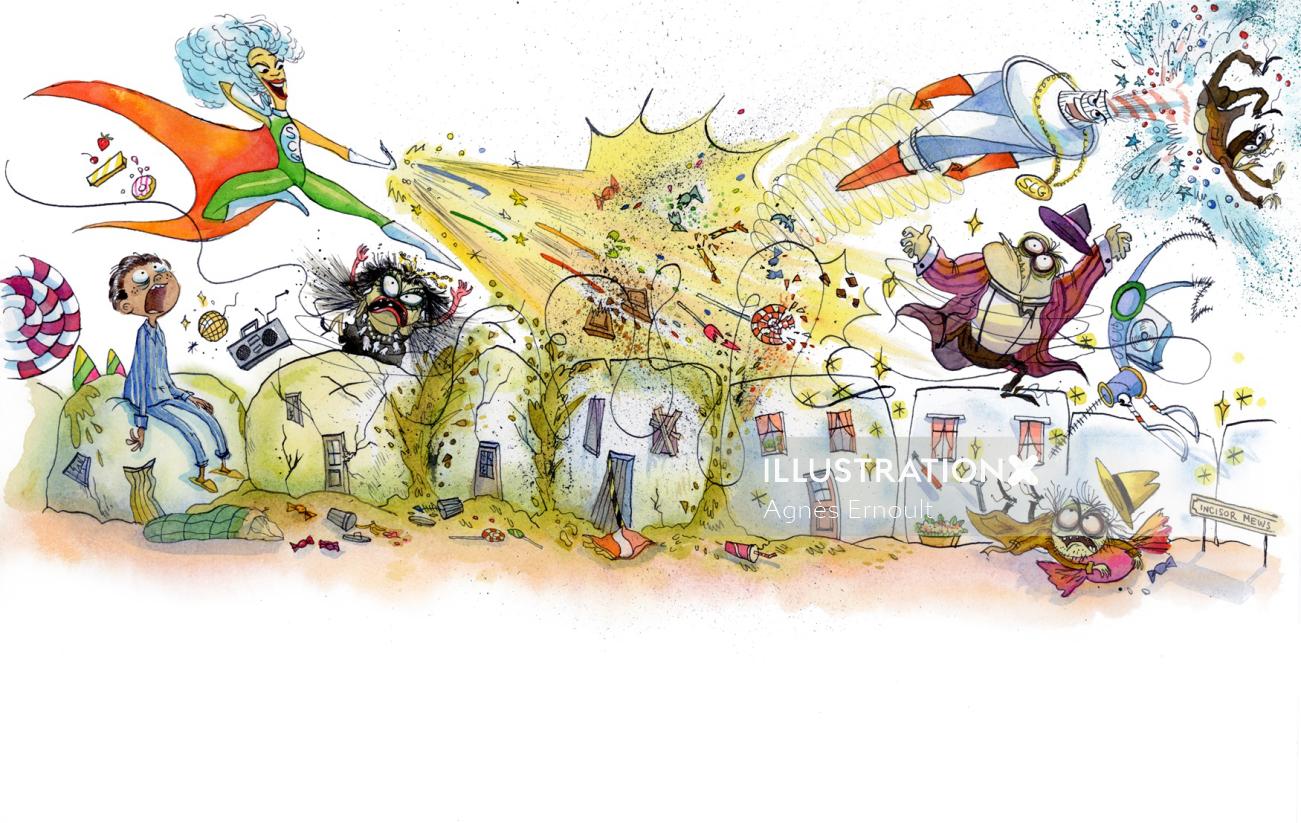This vibrant, hand-drawn illustration, potentially CGI-augmented but retaining a distinctly handcrafted feel, depicts an intense superhero battle scene set in a decrepit cityscape of small, dirty houses. At the center is a hero woman with striking blue curly hair, a green jumpsuit, orange cape, and yellow skin, her left arm resembling a hook as she shoots explosive energy. Opposed to her is a quirky, toothpaste-shaped character in a purple suit and hat, with large bug eyes and gray skin, retaliating with streams of toothpaste-like substance aimed at surrounding criminals. 

The chaos unfolds in a densely packed, busy scene with numerous small homes, some with multiple doors. A young boy, seated on one of the houses, looks on in distress, amplifying the scene's urgency. Meanwhile, in the far upper right corner, another creature is seen being ejected, possibly from an explosion or a cannon blast. The artwork is marked with a subtle watermark reading "Illustration X Agnes Arnault,” blending into the dynamic backdrop of the illustrated chaos.